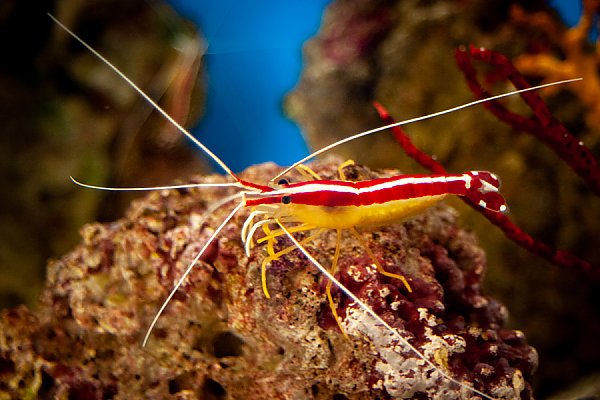This highly detailed and vibrant underwater photograph showcases a remarkably colorful shrimp resting horizontally on ocean coral. The shrimp's body features a striking color pattern: a broad white stripe runs from its head to its red tail, which is adorned with white spots. The top of the shrimp is predominantly red, while its underside and multiple legs are yellow. The shrimp has five elongated white antennae extending from its head, which has black, protruding eyes. The front two legs are white, contrasting with the yellow hue of the remaining legs. Beneath the shrimp's tail, there appears to be a red, tube-like structure, which could be part of the coral or the shrimp's anatomy. The background of the image fades into a blurred mix of brown, red, and white coral with a blue ocean backdrop, suggesting an underwater scene or possibly an aquarium. The shrimp's vibrant and elaborate coloring makes it appear almost surreal, yet it remains a true depiction of marine life.